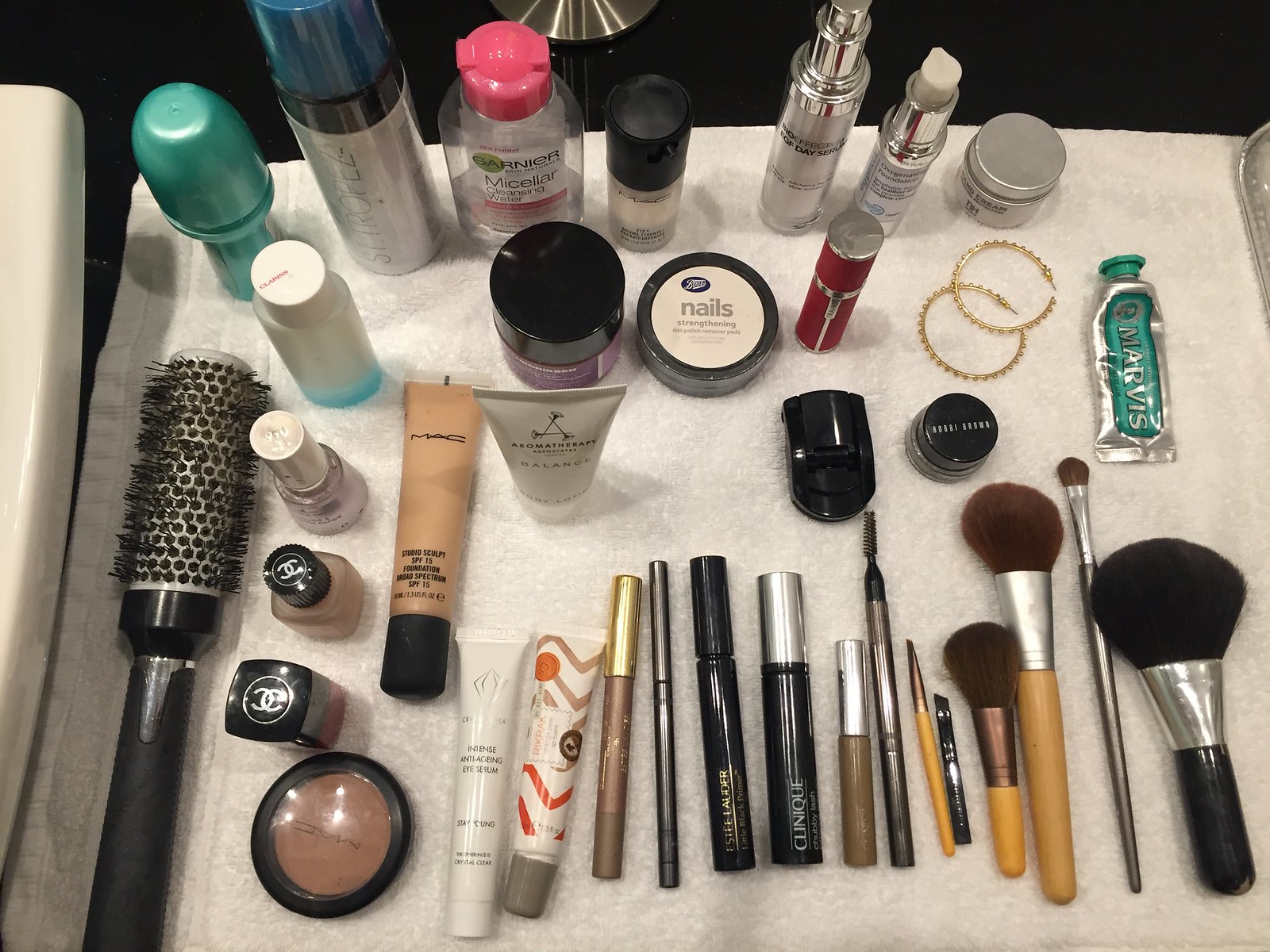This detailed photograph captures an assorted collection of beauty products meticulously arranged on a textured cloth, suggesting it might be set within a beauty parlor or shop. Dominating the bottom left corner is a cylindrical hair curler, characterized by its black "club-like" design reminiscent of medieval weaponry but intended for hair styling. This curler features a multitude of small black cylindrical bristles and a long black handle. Over on the bottom right are multiple foundation brushes. One is large, black, and bushy, while several others are slimmer with fine brown bristles and sleek beige handles. Centered on the bottom of the image, eyeliner products intended for enhancing the darkness of eyelashes are visible. Scattered across the top of the table are various mysterious liquid containers and spray bottles, adding to the array of beauty tools. A pair of elegant golden earrings adorns the top right corner, adding a hint of glamour and sophistication to the display.